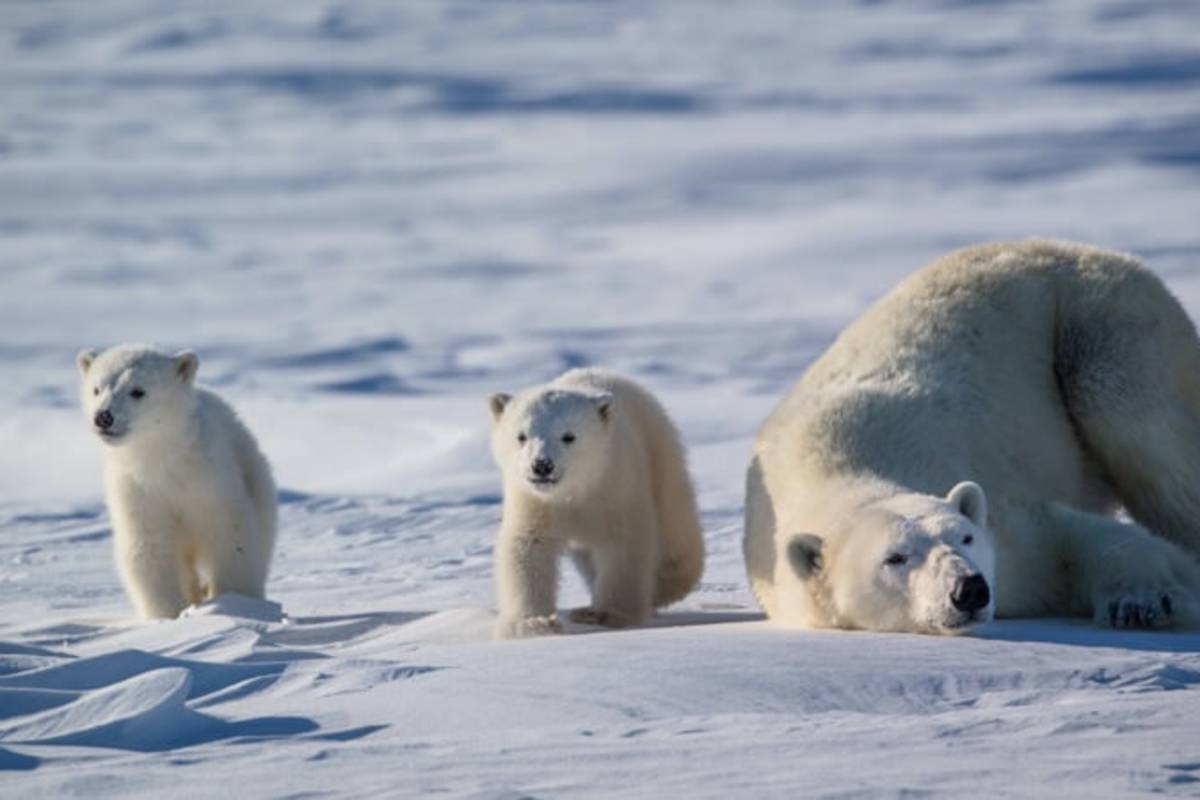In this captivating photo, we see a family of polar bears against the backdrop of a seemingly endless, bright expanse of snow. The scene features a mother bear and her two adorable cubs. The mother polar bear appears exhausted, lying with her head down and her back end raised, as if she’s landed in that position for comfort. The snow surrounding them is brilliantly white with a bluish tinge, enhanced by the clear, sunny day that casts distinct shadows.

The two cubs are beside their mother, each striking a different pose. One cub gazes intently into the distance, possibly curious about its surroundings or considering a wander. The other cub, equally cute, seems to be looking directly at the camera, perhaps aware of the photographer’s presence. Despite the cubs' alertness, the mother bear seems entirely unconcerned, content in her repose. This serene moment captures the simple beauty and gentle dynamics of a polar bear family in their natural, snowy habitat.